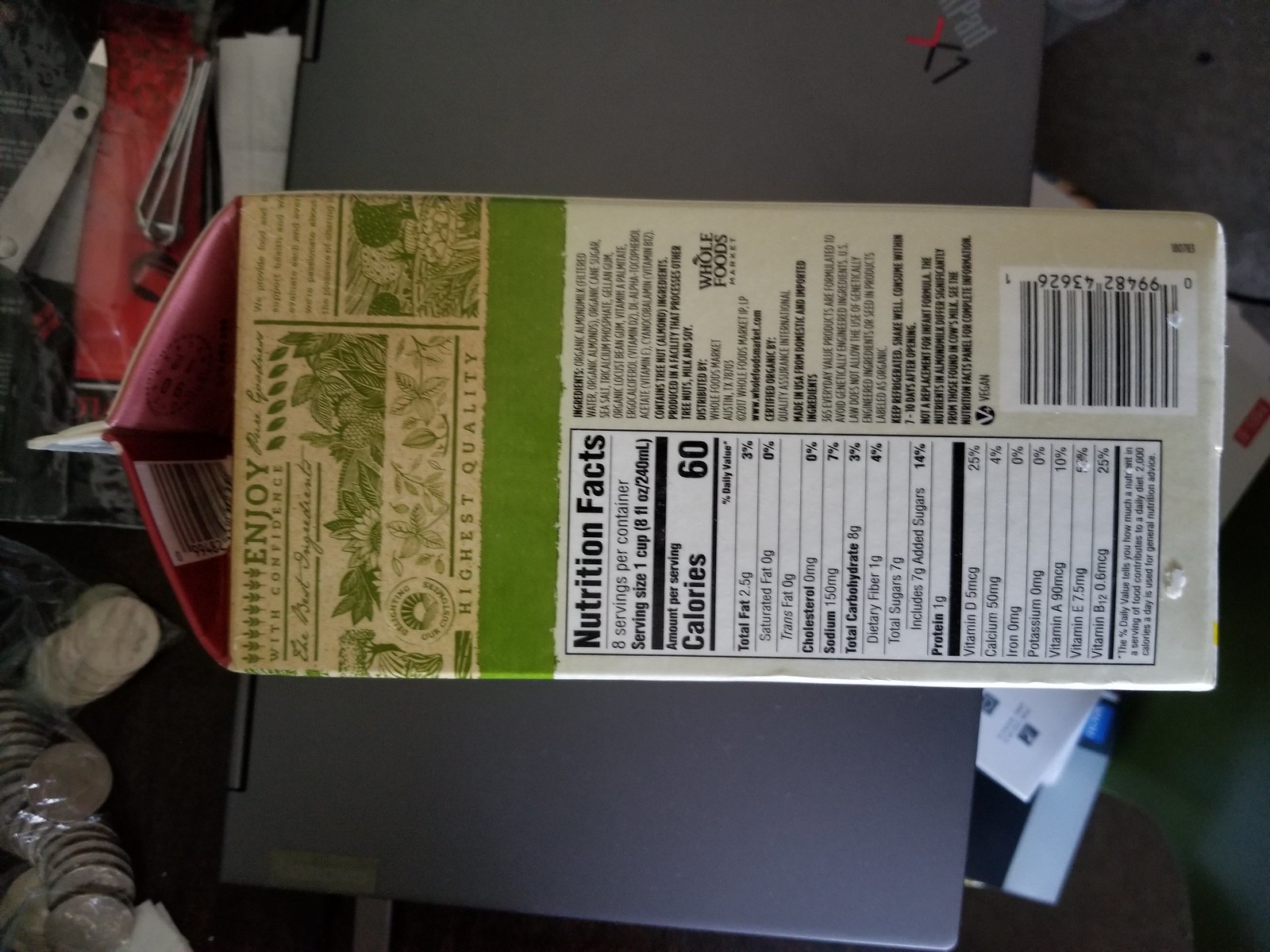The photograph depicts a vibrant, rectangular carton of food, reminiscent of a milk carton, positioned horizontally within the indoor frame. The carton features a peaked top with a characteristic ridge, similar to that of a traditional milk container. The body of the carton is adorned with a striking palette of red, gold, green, and tan hues. 

The side facing the camera prominently displays a white nutrition label and a UPC barcode in black type. At the top of this side, a rectangular section with a gold background and green graphics captures attention, containing legible text that includes the words "enjoy" and "highest quality." The barcode is situated at the bottom of the carton, which indicates a calorie count of 60 as per the nutrition facts. Additionally, the back of the carton bears the Whole Foods label.

The carton is placed horizontally across a laptop keyboard and a small pile of coins, which provides a sense of scale and context to the overall scene. The arrangement accentuates the detailed design and informative aspects of the carton, highlighting its packaging and branding elements in a everyday setting.